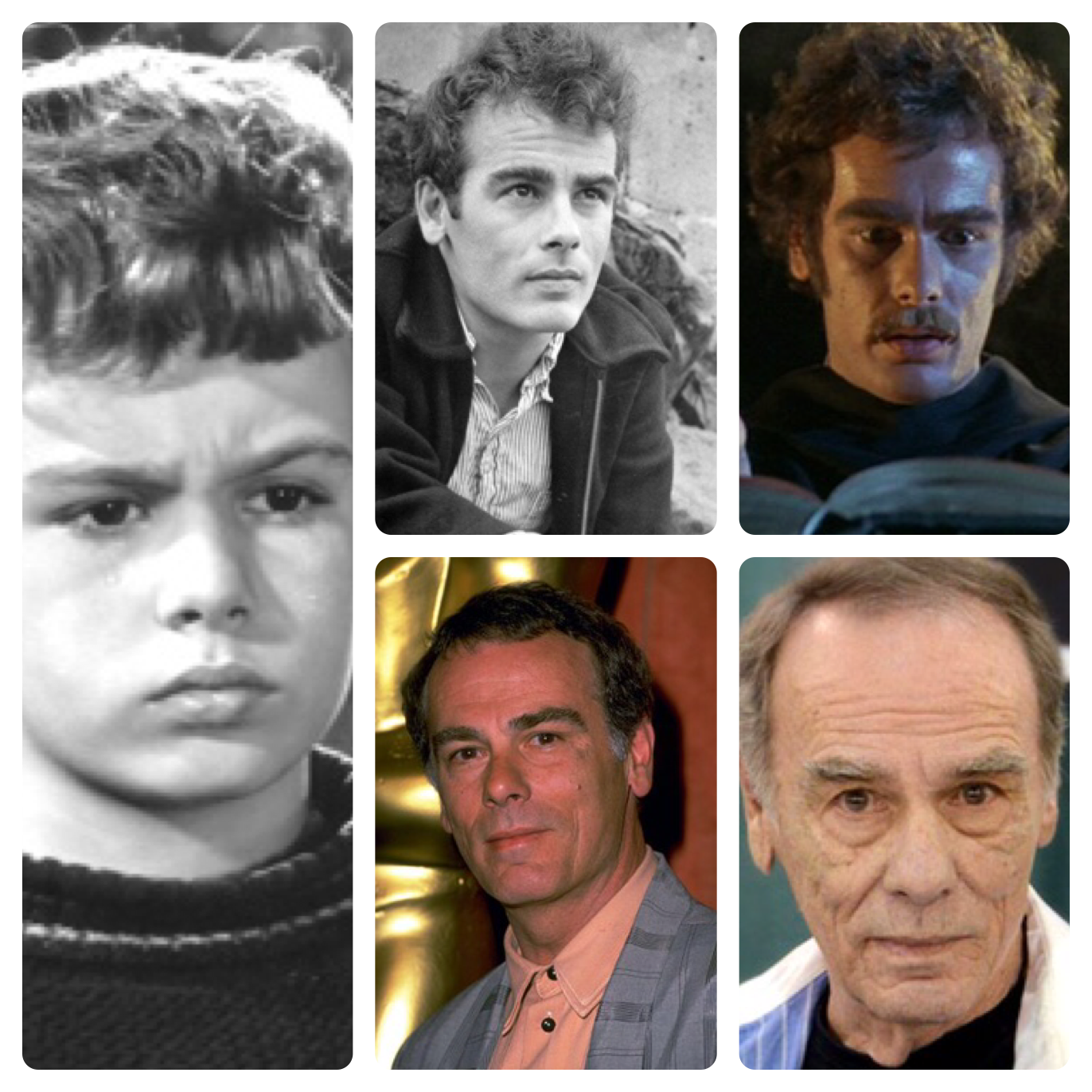The image is a collage of five photographs chronicling the same man's life at various stages. On the far left, occupying a third of the frame, is a black and white photo of him as a young boy, with short hair, a serious expression, and wearing a black sweater. Moving to the middle, the top photo shows him slightly older in another black and white shot, now with curly hair, presumably in a leather jacket and a white pinstripe shirt, maintaining a serious demeanor. Below it, an older version of him appears in a color photograph, standing beside an Oscar statuette in a formal peach-colored shirt and gray suit, indicating a significant career achievement. In the upper right, he appears in his 30s with curly hair that poofs out, a mustache, and a surprised look on his face, dressed in a black sweater. Finally, the bottom right photo, also in color, depicts him as an elderly man with thinning, graying hair, more wrinkles, and a serious expression, dressed in a dark shirt with a white jacket.